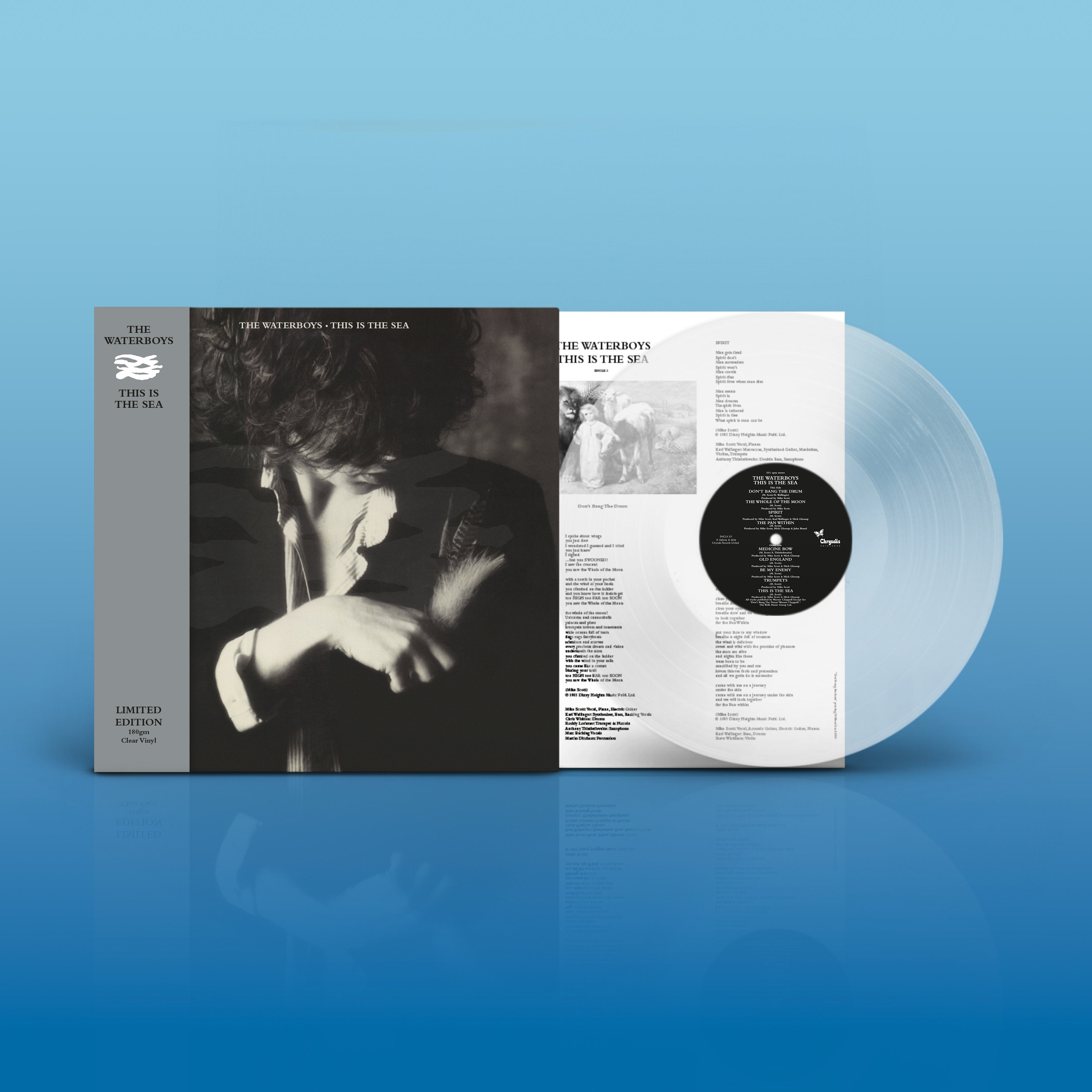This photograph captures a visually striking presentation of a limited edition vinyl record and its packaging. Set against a background that transitions from a dark to a lighter shade of blue, the record itself is semi-transparent, exhibiting a unique cloudy appearance. Its center is marked by a black label with fine white text that is somewhat hard to decipher. The album cover prominently features a black and white photograph of a person with long hair, obscuring most of their face except for the tip of their nose and lips, as they face right, wearing a dark jacket. At the top of the cover in bold white lettering, it reads "The Water Boys." Beneath that to the left, a vertical gray bar contains additional album details: "The Water Boys" in black at the top, a small white logo, the title "This is the Sea," and a declaration of "Limited Edition" near the bottom. A hand holding a feather reaches up towards the front pocket of the person's clothing. The album also appears to include an insert that likely contains the song lyrics.